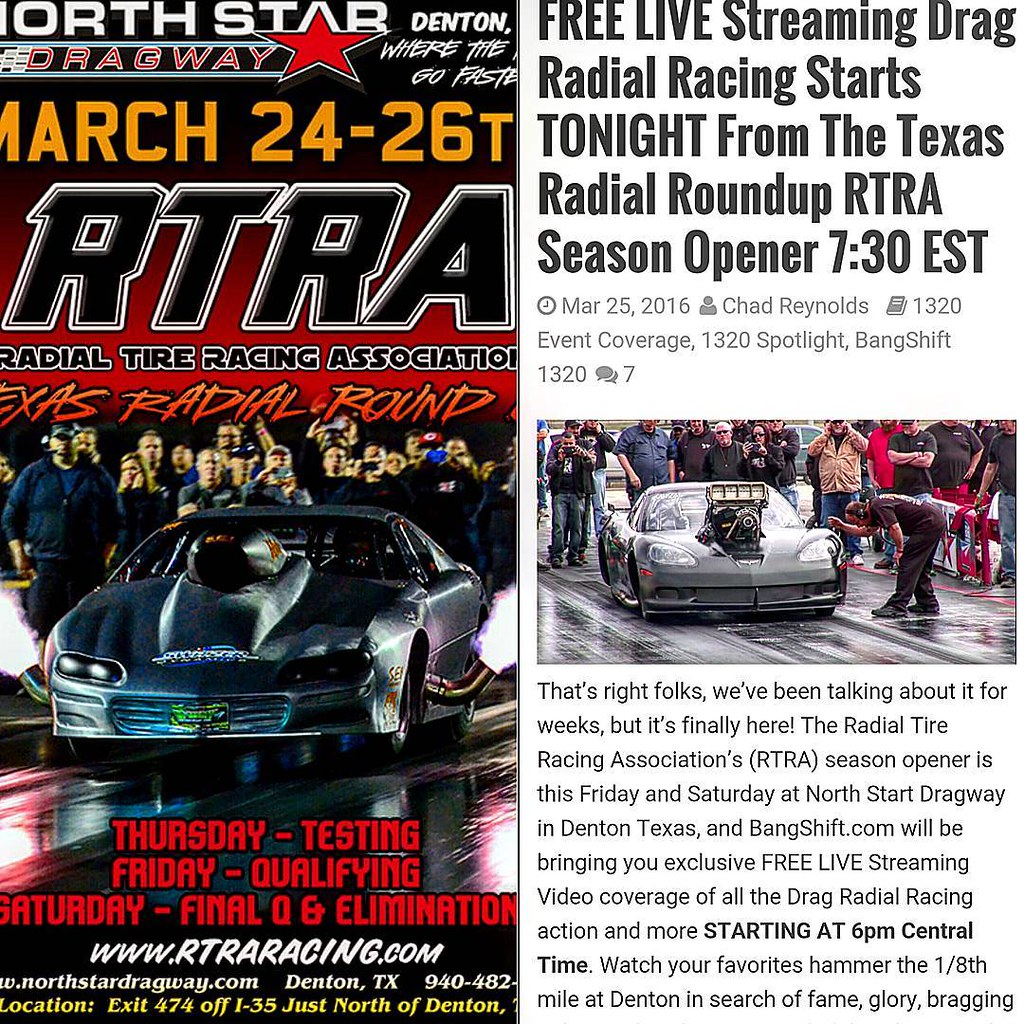The image is a split promotional poster and newspaper article for the Radial Tire Racing Association (RTRW) Season Opener at North Star Dragway in Denton, Texas, scheduled from March 24 to 26. The left side of the poster prominently displays "North Star Dragway" with a red star, alongside event dates. Centered on this side is a dynamic photo of a black race car with exhaust pipes emitting flames, surrounded by numerous spectators capturing the thrilling moment. Event details below the car list Thursday testing, Friday qualifying, and Saturday final and elimination rounds, with an address and the website www.rtdraracing.com.

On the right side, an article titled "Free Live Streaming Drag Racing Starts Tonight from the Texas Radial Roundup RTRA Season Opener 7:30 EST" highlights the event's coverage. Accompanying this section is another image of a gray race car with a prominent engine, surrounded by spectators, further enhancing the excitement. The article underneath informs readers about the event's exclusive live stream on bankswitch.com, starting from 6 p.m. Central Time, providing in-depth coverage of the action-packed drag radial racing.